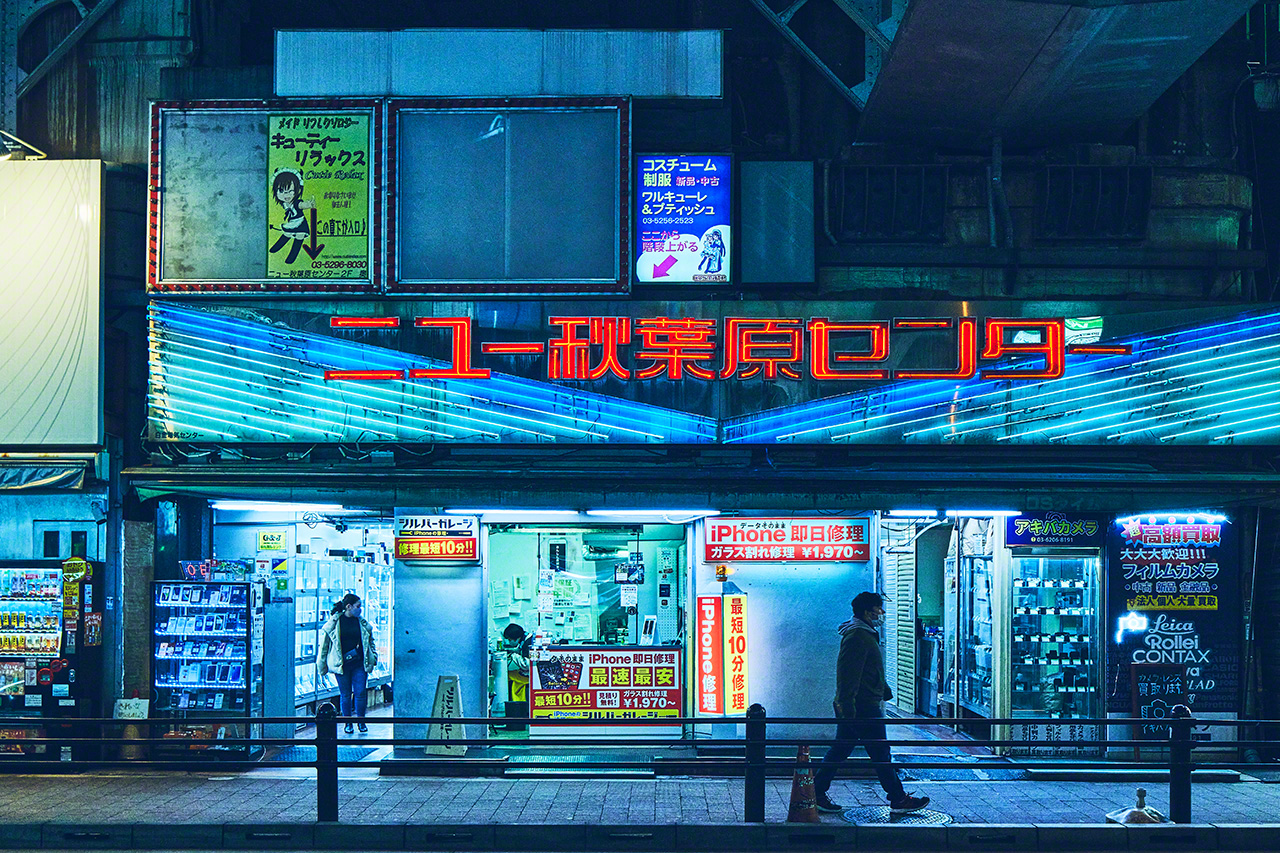This nocturnal photograph captures a futuristic, sci-fi postmodern phone store in Japan. The image, reminiscent of a Google Maps street view, showcases a vivid scene illuminated by the store’s dramatic lighting. The store, named "Mew Santa," beckons with large red neon text, standing as a single-story establishment amidst a row of similarly lit mobile shops. Each shop window is adorned with advertisements, prominently featuring an iPhone available for 1,970 yen, amidst a variety of other electronic products. The bustling facade includes vending machines, one glowing a distinct blue, contributing to the scene’s futuristic ambiance. A woman is captured leaving the illuminated store while a man walks along the metallic-fenced sidewalk, heading to the right side of the frame. The overall composition of the photograph combines everyday commerce with an otherworldly aesthetic, reflecting the vibrant, tech-savvy culture of nocturnal Japan.